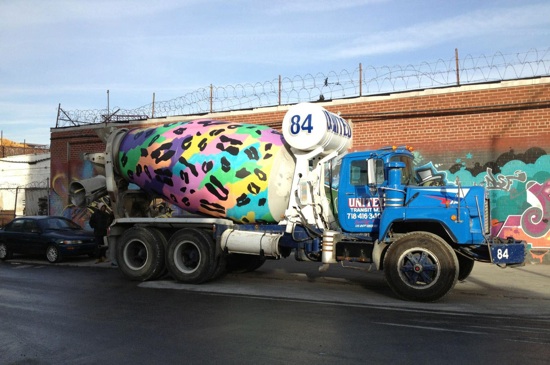This is a vibrant and detailed color photograph depicting a cement mixer truck parked in front of a red brick building adorned with graffiti and topped with barbed wire. The truck's cab is painted blue with the words "United Transit" inscribed on its side, along with an unreadable phone number. The main feature of the truck—the cement mixer barrel—is a striking display of artistry, covered in splashes of bright pink, green, purple, blue, yellow, and orange, with an overlay of white blotches and a leopard print pattern. The white tank situated between the cab and the mixer barrel bears the number 84. This industrial vehicle is positioned on the side of the road, near a dark colored car, with a person barely visible between them. In the setting, there's a mix of urban elements including a wire fence and chain link fence, adding to the bustling atmosphere captured in the image.